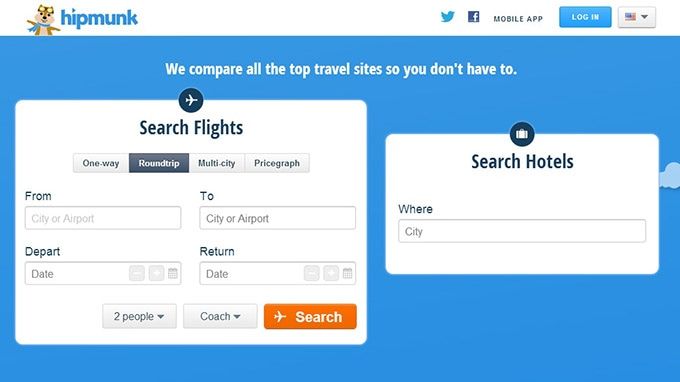The image depicts the login screen of the Hipmunk travel app, which includes icons for Twitter, Facebook, and the American flag. Users have the option to search for airline flights, with choices for one-way, round-trip (selected), or multi-city itineraries. Input fields for departing and returning city or airport names are present, along with drop-down calendars for selecting travel dates. There are also options to specify the number of travelers (defaulting to two) and the travel class (coach by default) using drop-down menus. An orange button labeled "Search" in white text is situated to the right. Additionally, there is a section to search for hotels with a specified city, indicated by a text field. The background features a blue sky with a single cloud on the right side, contributing to a serene and welcoming atmosphere. The app prominently displays various social media icons, with Facebook and Twitter appearing multiple times, alongside others like Instagram and Snapchat.